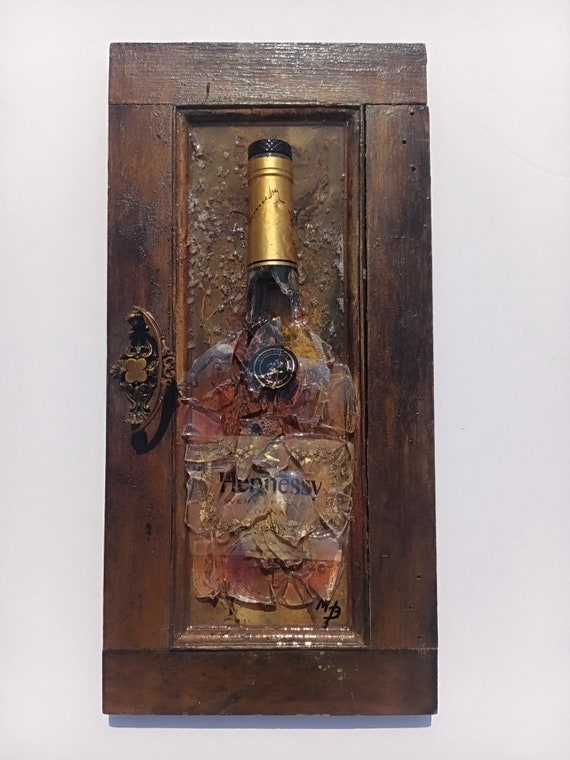The image features a detailed wooden display case made of aged, dark-stained wood with a distinctive bronze catch on the side. Although it's unclear whether the case actually opens, the sophisticated design gives it the appearance of having a door. This display case is mounted against a light gray or white wall. Inside the case, a bottle of Hennessy Cognac is prominently featured. The bottle remains sealed with its golden foil band intact around the neck, but the rest of the bottle is shattered and meticulously reassembled, with noticeable gaps between the glass pieces, allowing the label "Hennessy" to remain legible. The artist's initials, "MP," are discreetly placed at the bottom, suggesting a thoughtful, artistic interpretation. This unique art piece presents a striking contrast between the pristine condition of the bottle's neck and the shattered chaos below, all encased within the rustic wooden frame.